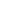The image captures a distant city skyline shrouded in a thick orange-brown haze, creating a mysterious and dramatic atmosphere. The sky is dominated by a flat, sepia-toned gradient with a brighter orange streak across the middle, suggesting either a golden sunset or an unusual weather phenomenon. The tops of approximately 15 skyscrapers pierce through the haze, their blocky and box-shaped forms highlighted by sunlight reflecting off their surfaces. These buildings are organized in clusters: the left side of the image shows a tightly-packed group of tall skyscrapers, the center has slightly shorter buildings clustered together, and the right side features more widely spaced, shorter structures. At the very bottom of the image, some tree canopies peek through the shadows, adding a touch of dark green to the otherwise monochromatic scene. Despite the haziness, the buildings can be clearly distinguished, though they lack any visible branding or distinctive architectural details. This evocative image leaves viewers questioning whether they are witnessing a natural phenomenon like a sunset or a scene affected by atmospheric conditions similar to a dust storm or heavy smog.